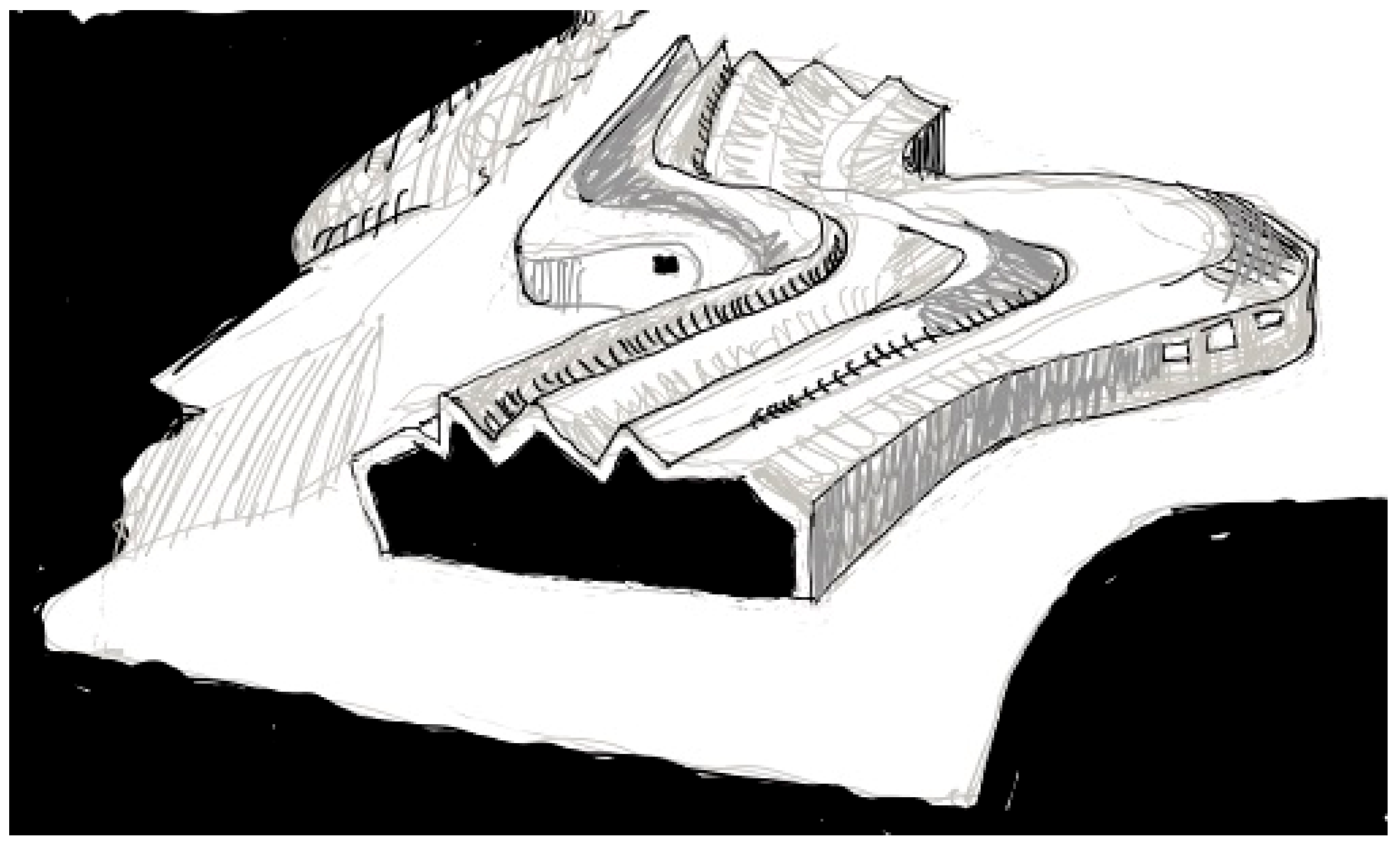This black and white, hand-drawn, pen and ink sketch depicts an amorphous, building-like structure with grooved lines and an S-shaped form. The structure features three small windows on the right curve and ends abruptly in a black, cut-off maw, indicating an entryway reminiscent of a tunnel's opening. The image includes texture details, with scribbled lines along the top and a sense of white space surrounding the main structure, giving it a bold outline. The overall appearance suggests an abstract concept of a possibly underground or partially covered tunnel system, with a mix of organic and industrial design elements.